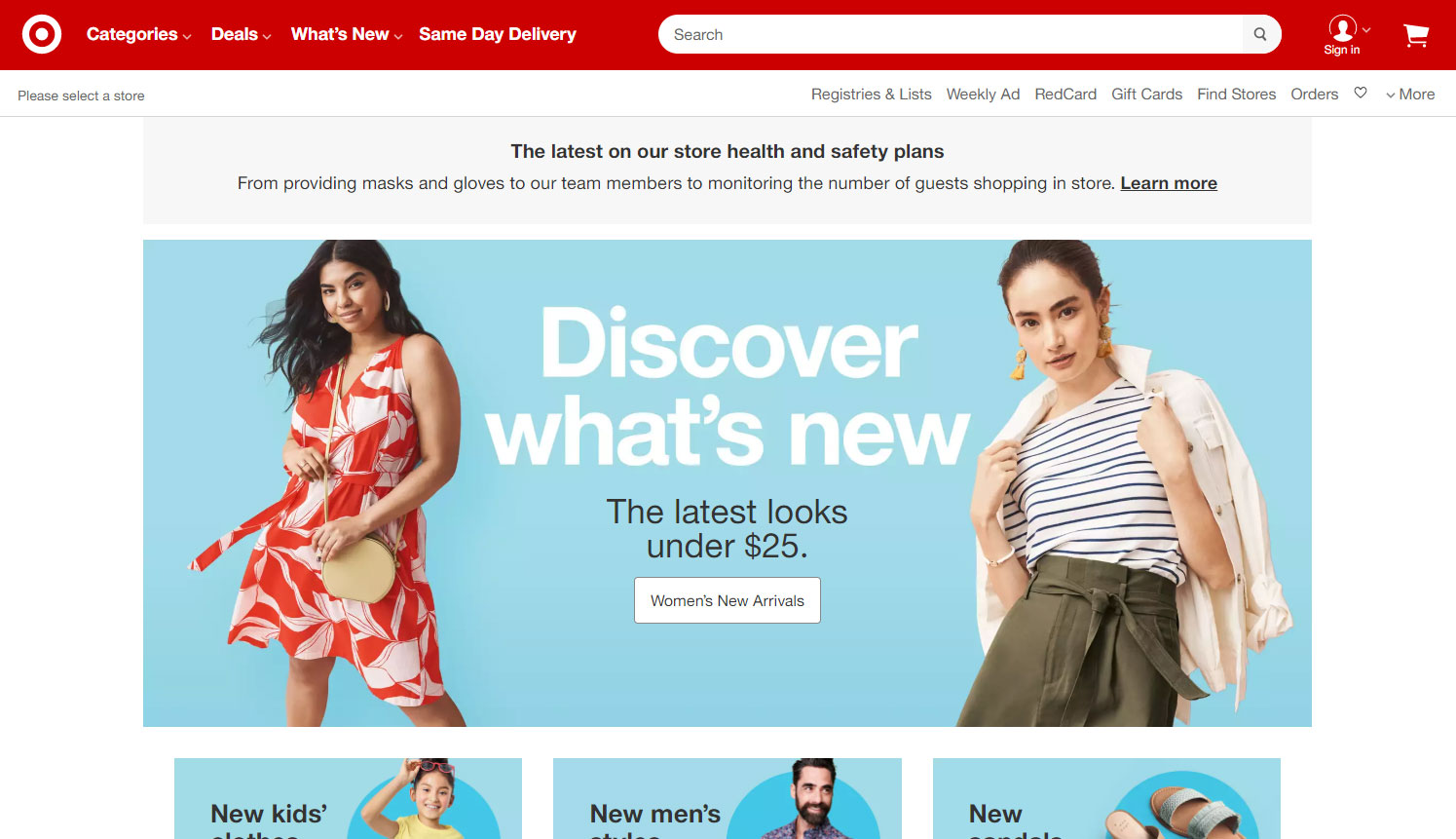This detailed screenshot of the Target web page features several design elements and sections aimed at enhancing user experience. At the top, a prominent horizontal red bar stretches across the screen, providing a cohesive brand identity. In the top left corner, the recognizable Target logo is displayed, followed by navigation options that include "Categories," "Deals," "What's New," and "Same Day Delivery." Adjacent to these, a search bar is centrally located, while to the right, user-specific options like "Sign In" and a shopping cart icon are present.

Directly below, a secondary, horizontal leather-textured menu bar offers additional navigational links such as "Registries and Lists," "Weekly Ad," "RedCard," "Gift Cards," "Find Stores," "Orders," and a "More" dropdown. An instructional prompt urging users to "Please select a store on the left" is visible, emphasizing the personalization of the shopping experience.

Prominently below this bar is a gray notification box highlighting the company's commitment to health and safety measures, including the provision of masks and gloves to team members and the regulation of guest numbers in stores. A "Learn More" link is included for further details.

Navigating further down, the page features a large, attention-grabbing blue advertisement with the headline, "Discover What's New: The Latest Looks Under $25." A gray button labeled "Women's New Arrivals" invites users to explore more.

Within the ad, two women are depicted showcasing trendy outfits. The woman on the left has an olive to medium brown skin tone, black hair, and wears a stylish red and white sundress cinched with a belt. The woman on the right appears to be of Asian descent, characterized by pale skin, yellow earrings, and a chic ensemble consisting of a white striped shirt paired with a grayish pencil skirt.